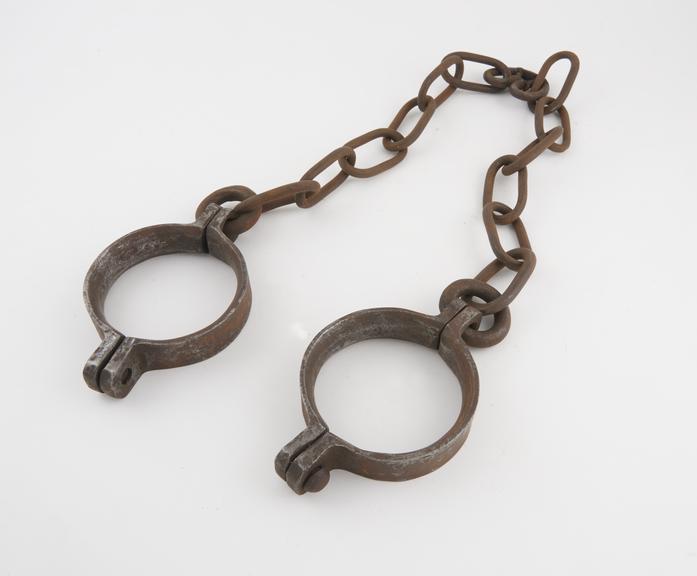The photograph showcases a pair of vintage leg irons lying against a pure white background. The shackles, which encircle the ankles, are conspicuously rusted to a dark, foreboding red-brown hue. One of the shackles has a bolt inserted, while the other is missing its bolt. They are connected by a long, heavy, equally rusted chain, comprising approximately 15 links, allowing enough length for movement. The metal of the shackles, though heavily corroded, hints at its original gray color beneath the layers of rust. The overall composition of the image places the shackles below the center, pointed towards the left, creating a stark and solemn visual on the pristine white surface.